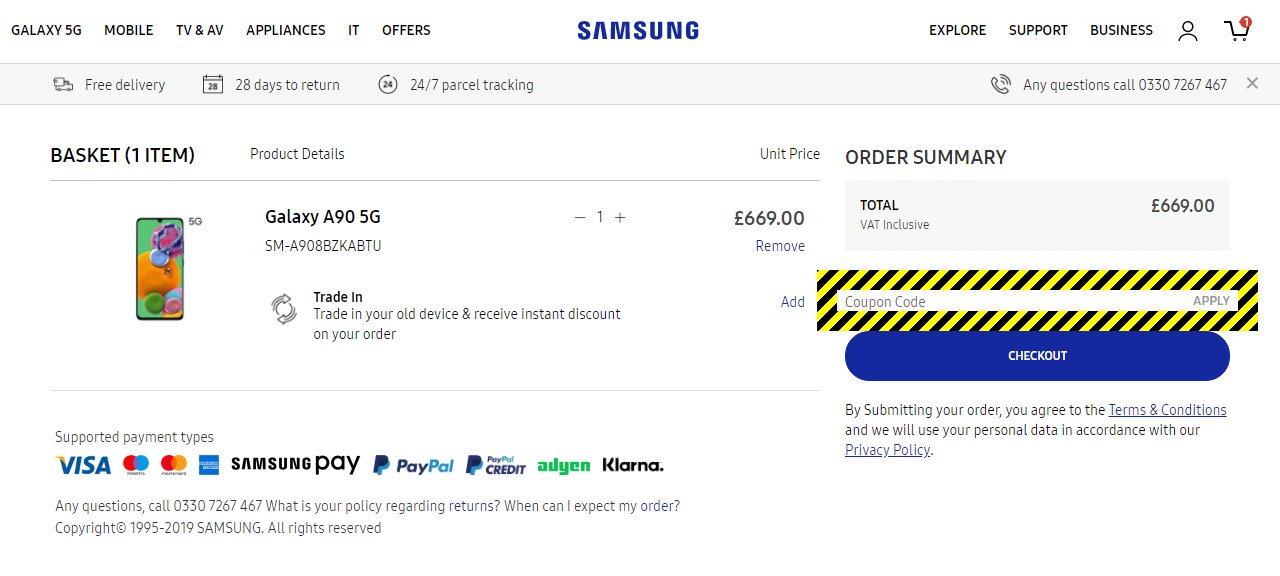A detailed caption for the image in question could read:

"This screenshot captures a page from the Samsung website. Prominently displayed at the top center is the 'Samsung' logo. To the upper left, there are multiple navigational tabs that users can select, labeled 'Galaxy 5G,' 'Mobile,' 'TV & AV,' 'Appliances,' 'IT,' and 'Offers.' In the upper right corner, additional options are available including 'Explore,' 'Support,' and 'Business,' alongside a profile icon and a shopping cart icon, the latter of which shows a notification with the number '1.' 

The shopping cart interface, located more towards the left, includes a 'Basket' section showing 'one item' with accompanying 'product details.' The primary featured item is an image of a smartphone, specifically the 'Galaxy A95G,' priced at 669 euros. Within this interface, there is a designated area for entering coupon codes, notably highlighted by a thick rectangular border adorned with diagonal black and yellow stripes. Beneath this section, a prominent blue 'Checkout' button is displayed.

In the bottom left corner of the webpage, there is a list of supported payment methods which includes Visa, MasterCard, Samsung Pay, PayPal, and Klarna. Below the list, a phone number is provided for any policy-related queries."